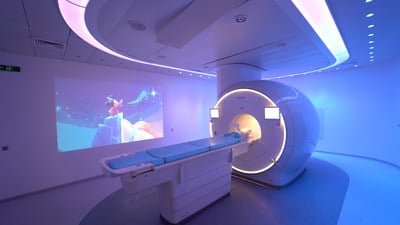This detailed photograph depicts a modern medical imaging room designed for cancer screening, featuring a sophisticated tube-like imaging machine. The room is strikingly illuminated in blue, with an oval or circular light installation on the ceiling, adding to its modernistic, almost futuristic ambiance reminiscent of a Star Trek set. The machine itself is large and round, equipped with lights and monitors on either side. At its foot lies a mechanized bed with a blue cushion that slides seamlessly into the machine, designed to accommodate patients comfortably during the procedure.

Adding an unexpected touch to the clinical environment, a Disney movie, seemingly a Mickey Mouse film, is projected onto one of the walls. This projection, likely intended to relax patients, especially children, offers a whimsical contrast to the high-tech setting. The floor and ceiling are uniformly gray, enhancing the room's sleek and sterile appearance.